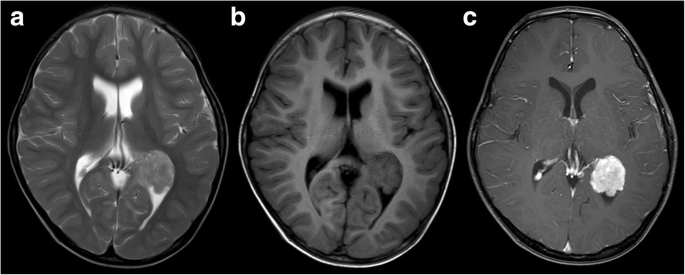The image displays three horizontal brain scans labeled A, B, and C from left to right, each set against a stark black background. Scan A predominantly features a dark gray brain with notable white regions centrally located, including two symmetrical, upside-down sock-like structures and smaller white patches beneath them. Scan B is characterized by an overall darker appearance where the central white areas seen in scan A are replaced with black spots, maintaining the shape but in a darker hue. Scan C, predominantly gray, exhibits less detailed contrast with a prominent white circle at the bottom right, suggesting a mass or potential brain tumor, differing from A and B. The brain scans appear consistent in shape and structure, potentially representing the same brain, but differing in the highlights of various internal features possibly reflecting different imaging techniques or aspects of the same condition.